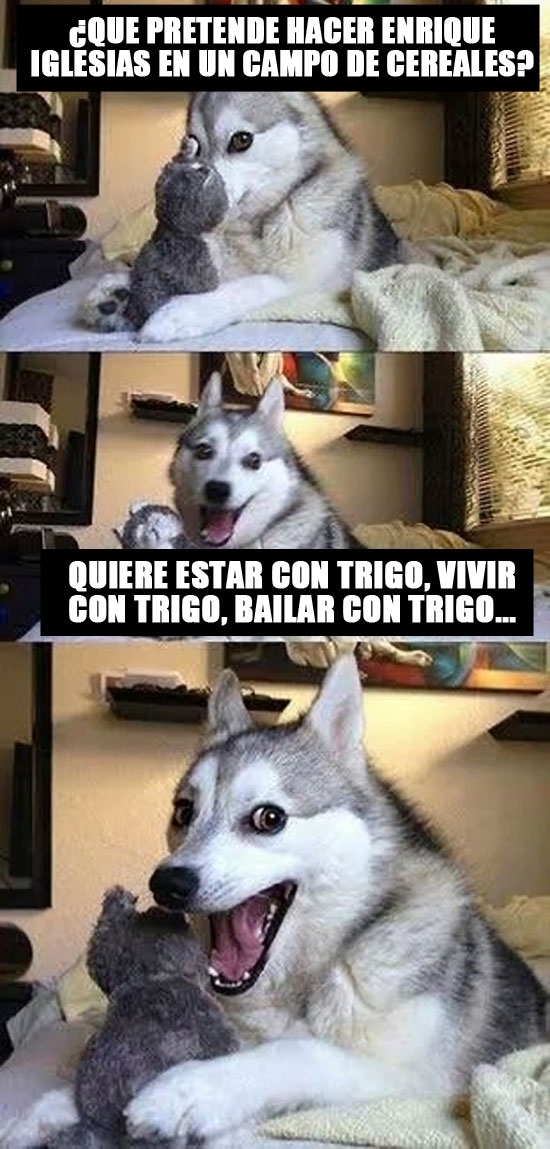The image is a vertical three-panel meme featuring a husky dog playing with a stuffed toy that looks like a dark gray teddy bear. The dog has distinct markings: a white nose, dark black eyes, and a mix of gray and white fur on its head, back, and paws. 

In the first panel, the husky is lying on a light gray bed, partially covered with a beige blanket, while holding the stuffed toy close to its nose. There's a black banner with white text overlaid, reading, "Pretend a sad Enrique Iglesias en un campo de cereales."

In the second panel, the same dog is depicted in the same setting but with its mouth wide open, looking directly at the camera, displaying its large pink tongue in a happy expression. The caption is similarly displayed on a black banner with white text, positioned below the image, saying, "Quiere estar con trigo, vivir con trigo, bailar con trigo."

The third and final panel shows the husky continuing to hold the stuffed toy, now appearing even more excited, with its mouth open wider, still looking straight ahead. This panel has no text or captions, emphasizing the dog's joyful expression.